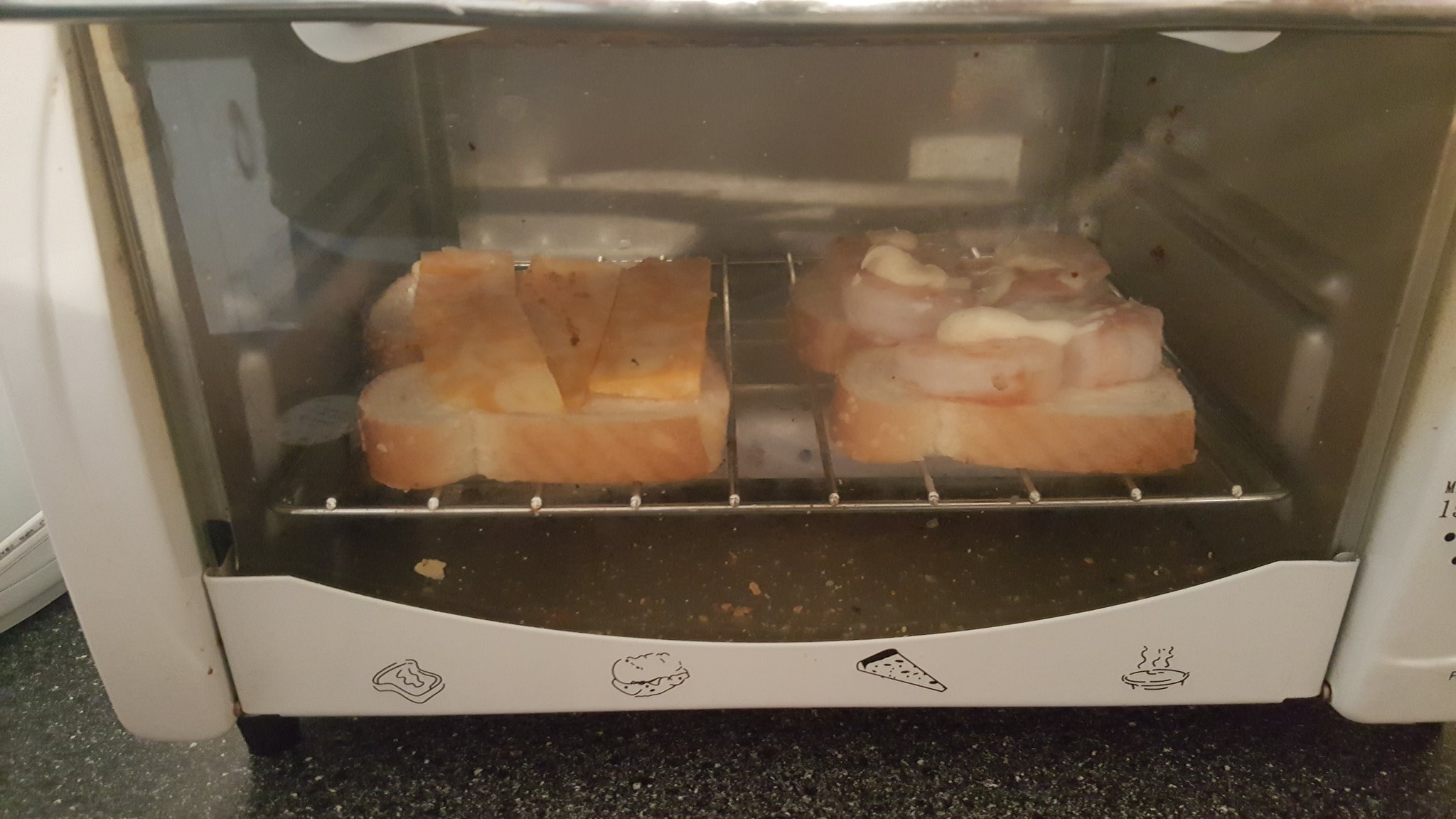This color photograph showcases the interior of a white metal countertop toaster oven, viewed through its glass door adorned with whimsical doodle icons of a sandwich, a slice of pizza, and a steaming pie. On a rack inside the oven, there are four open-faced sandwiches arranged in a 2x2 grid. Each sandwich consists of a thick slice of white bread. The two pieces on the left feature thick slabs of Colby Jack cheese, while the pieces on the right appear to be topped with a creamy white sauce and possibly shrimp. The door's bottom metal frame displays more playful doodles. A strip of granite countertop is visible at the bottom of the image. The entire scene is reflected faintly, revealing the shadow of the person who took the photo in the toaster oven's glass.